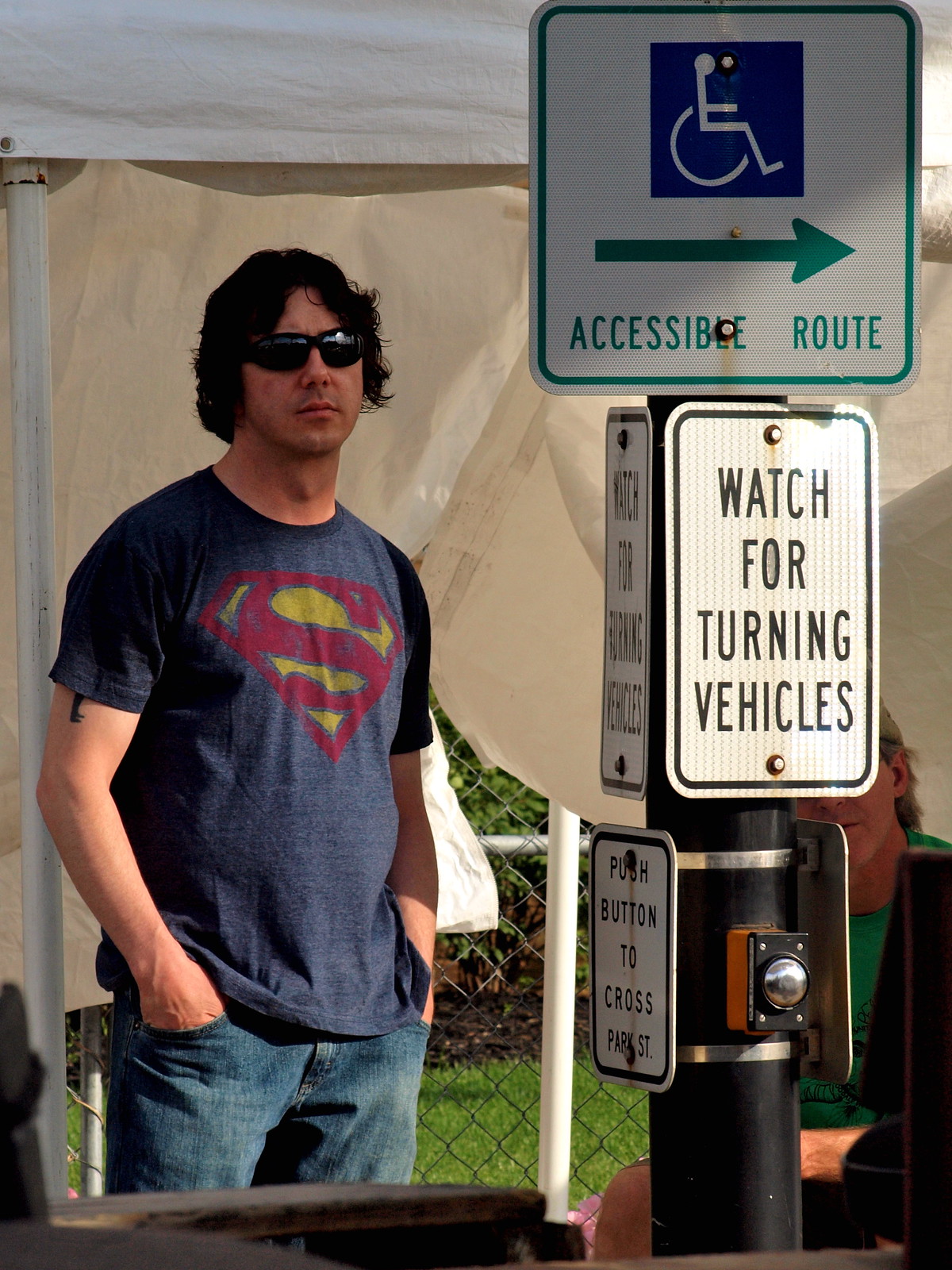The photograph captures a white man standing outside with a casual yet confident demeanor, looking directly at the camera. He sports long, slightly curly black hair that falls just past his ears and is parted in the center. His eyes are obscured by reflective, dark-colored sunglasses. His outfit consists of a dark blue Superman t-shirt featuring the iconic red 'S' symbol on a yellow diamond-shaped background and blue jeans. Both of his hands are casually tucked into his jeans pockets.

To the right of the man, there's a black metal pole adorned with several street signs. At the top, a white square sign with a green border and a blue and white handicap icon directs an accessible route to the right via a green arrow. Below it, a vertical rectangular sign reads "Watch for Turning Vehicles" in black text. Further down, there's a small sign indicating "Push button to cross Park Street," although part of the text is slightly obscured by rust. Attached to the pole is a silver and black pedestrian crosswalk button.

The background features a cream-colored tent with visible white poles, suggesting some kind of event or gathering. Behind the tent, there's a woman wearing a green shirt, partially obscured by the pole, presumably seated on a bench. The scene is set against a backdrop of grass and further hints of urban elements like a chain link fence, enhancing the outdoor atmosphere.